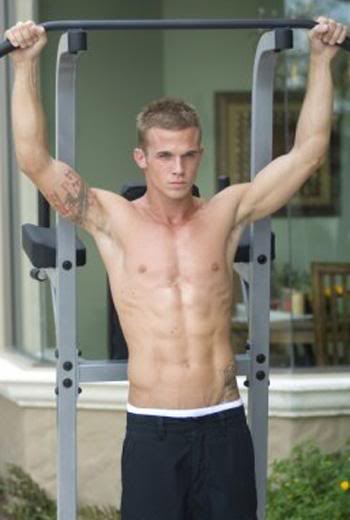A young man, estimated to be between 22 and 26 years old, is shirtless and wearing black shorts, lifts a barbell overhead. Though the weights on either end of the barbell are not visible, it's clear he is engaged in a weightlifting routine. He has a tattoo visible on his right bicep and maintains a neutral expression. Surrounding him at the lower corners of the image are green shrubs. Behind him, a window reveals the interior of a home, which features brown furniture, a brown-framed picture on the wall, and a brown table adorned with a white tablecloth. The walls inside the home are a light shade of green. Additionally, there is gym equipment in the background, suggesting the setting is an outdoor area with access to fitness apparatus used for various lifting exercises.